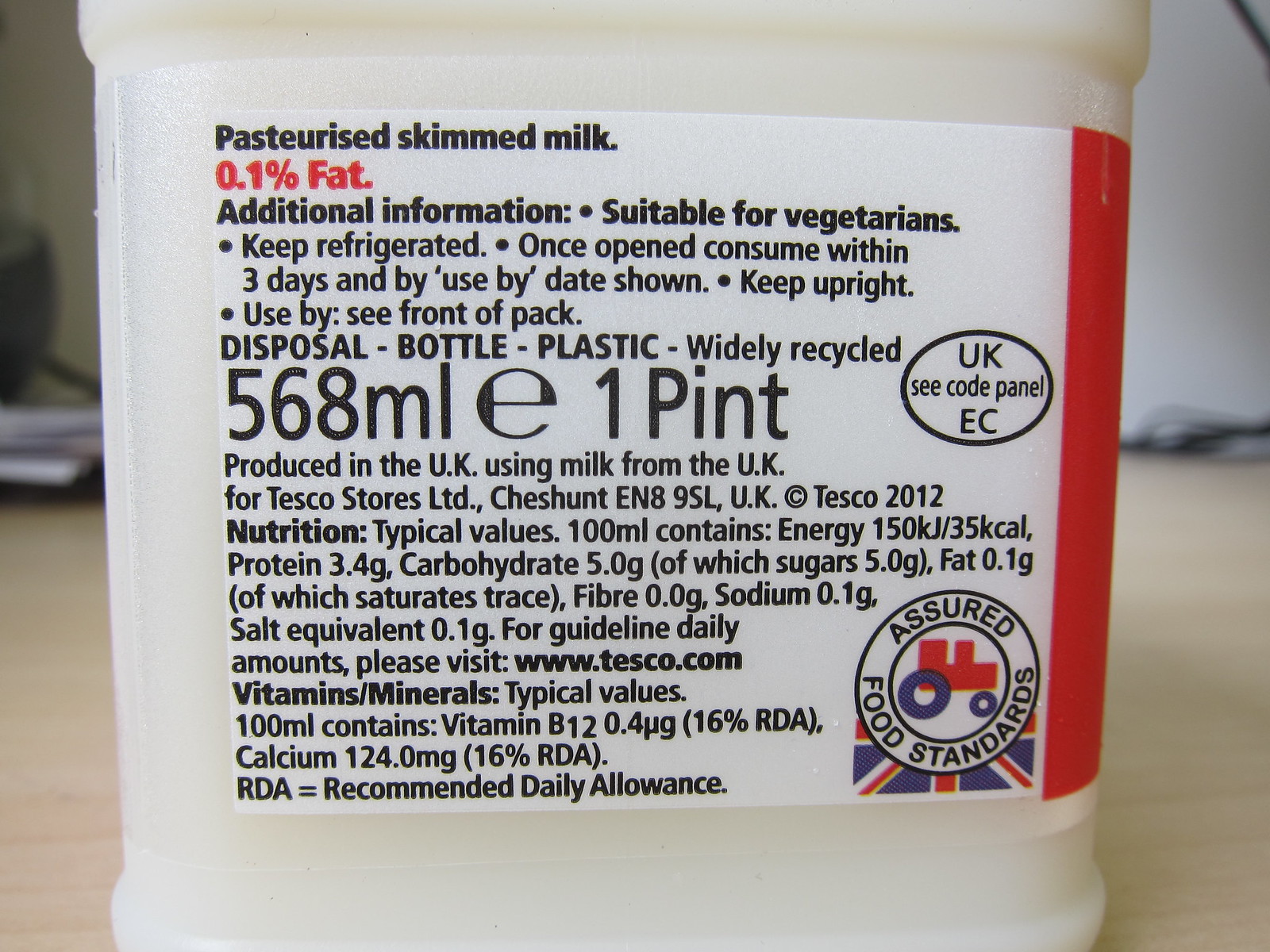The image displays the back label of a milk container, specifically for pasteurized skimmed milk with 0.1% fat. The container holds 568 milliliters, equivalent to 1 pint. Important storage instructions are provided: keep refrigerated, consume within three days of opening, and keep upright. The use-by date can be found on the front of the pack. The label also details that the product is suitable for vegetarians and is produced in the UK using milk from the UK for Tesco Stores Ltd. The container is made of widely recyclable plastic.

Nutritional information indicates that per 100ml, the milk contains 150 kilojoules of energy, 3.4 grams of protein, 5.0 grams of carbohydrates (all sugars), 0.1 grams of fat (trace amounts of saturates), 0.0 grams of fiber, 0.1 grams of sodium, and 0.1 grams of salt equivalents. It also includes 0.1 micrograms of Vitamin B12 (16% RDA) and 124.0 mg of calcium (16% RDA). There is a guideline daily amount link provided at www.tesco.com. Additionally, there are logos indicating compliance with UK food standards and assured food standards. The label also mentions the UKC code EC. 

Produced for Tesco in 2012, the detailed label emphasizes quality assurance and proper storage of the product.